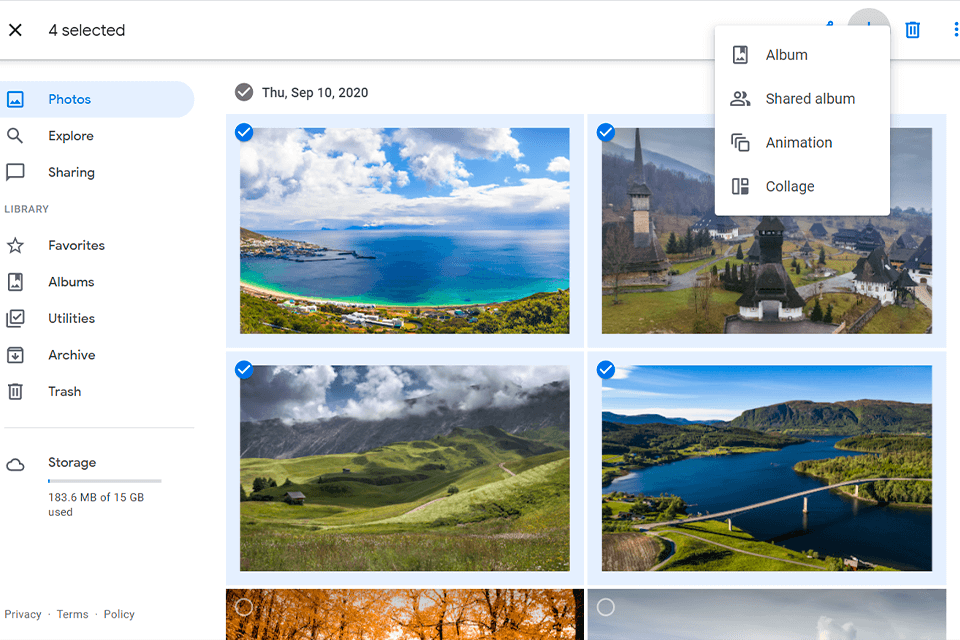In this image with a clean white background, there is a highlighted section labeled "X4" and a white box displaying various options: 'Album,' 'Shared Album,' 'Animation,' and 'Collage.' The date Thursday, abbreviated as 'THU,' along with 'SCP-10, 2020,' is prominently displayed. 

The image includes six photos: 
1. The first picture depicts a scenic view of water bordered by land and buildings. It is marked with a blue circle containing a checkmark.
2. The second picture features a collection of monuments and houses, also accompanied by a blue circle with a checkmark.
3. The third image captures a vast plain, a small house, distant mountains, and a cloudy sky, again marked with a blue circle and check.
4. The fourth photo shows a bridge spanning over water, with two landmasses on either side and cliff formations in the background, bearing the familiar blue circle with a checkmark.
5. The fifth and sixth pictures are not yet selected, indicated only by an outline of a circle.

To the left of the image, there is a contextual menu where 'Photos' is highlighted in light blue. Other options such as 'Explore,' 'Sharing,' 'Library,' 'Favorites,' 'Albums,' 'Utilities,' 'Archive,' 'Trash,' and 'Storage' are listed below. The storage section is lightly shaded in blue and indicates that 183.6 MB is used.